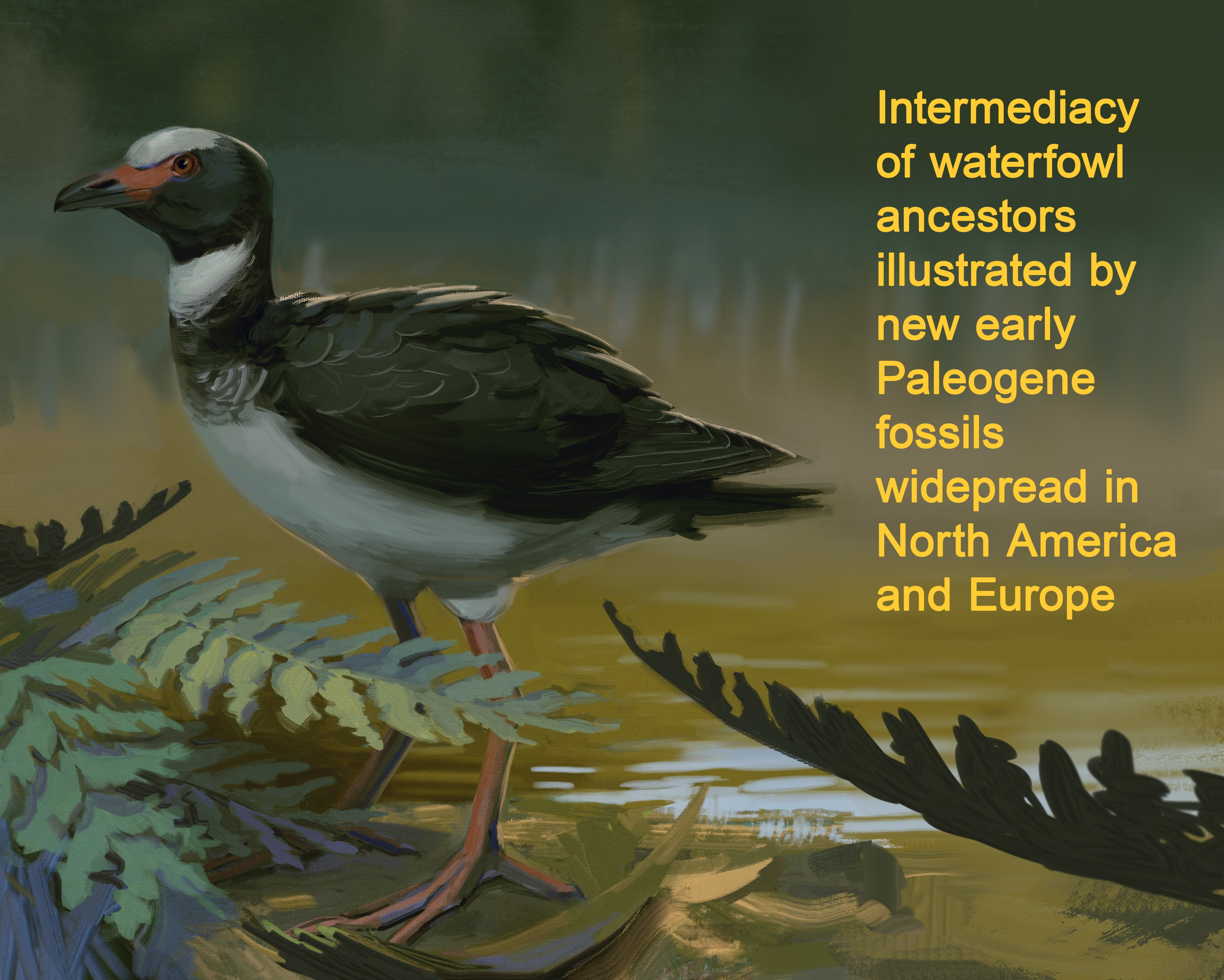This oil painting, slightly wider than it is tall, depicts a waterfowl standing on a misty shoreline with a murky, brackish water background that transitions from dark green to olive green and finally to a lighter green along the shore. The bird, potentially a duck, positioned on the left of the scene, has a distinctive appearance: white feathers adorn the top of its head and underbelly, while its eyes and head are tinged with red, and its beak is sharp, exhibiting an orange hue that darkens to black. Its neck and back are covered in black feathers. The bird stands on fairly long orange-webbed legs, partially obscured by green fern-like leaves that cover parts of its legs and extend from the ground. Additional silhouettes of ferns further emphasize the natural setting. In the right corner, in yellow font, the text reads: "Intermediacy of Waterfowl Ancestors, illustrated by new early Paleogene fossils widespread in North America and Europe."